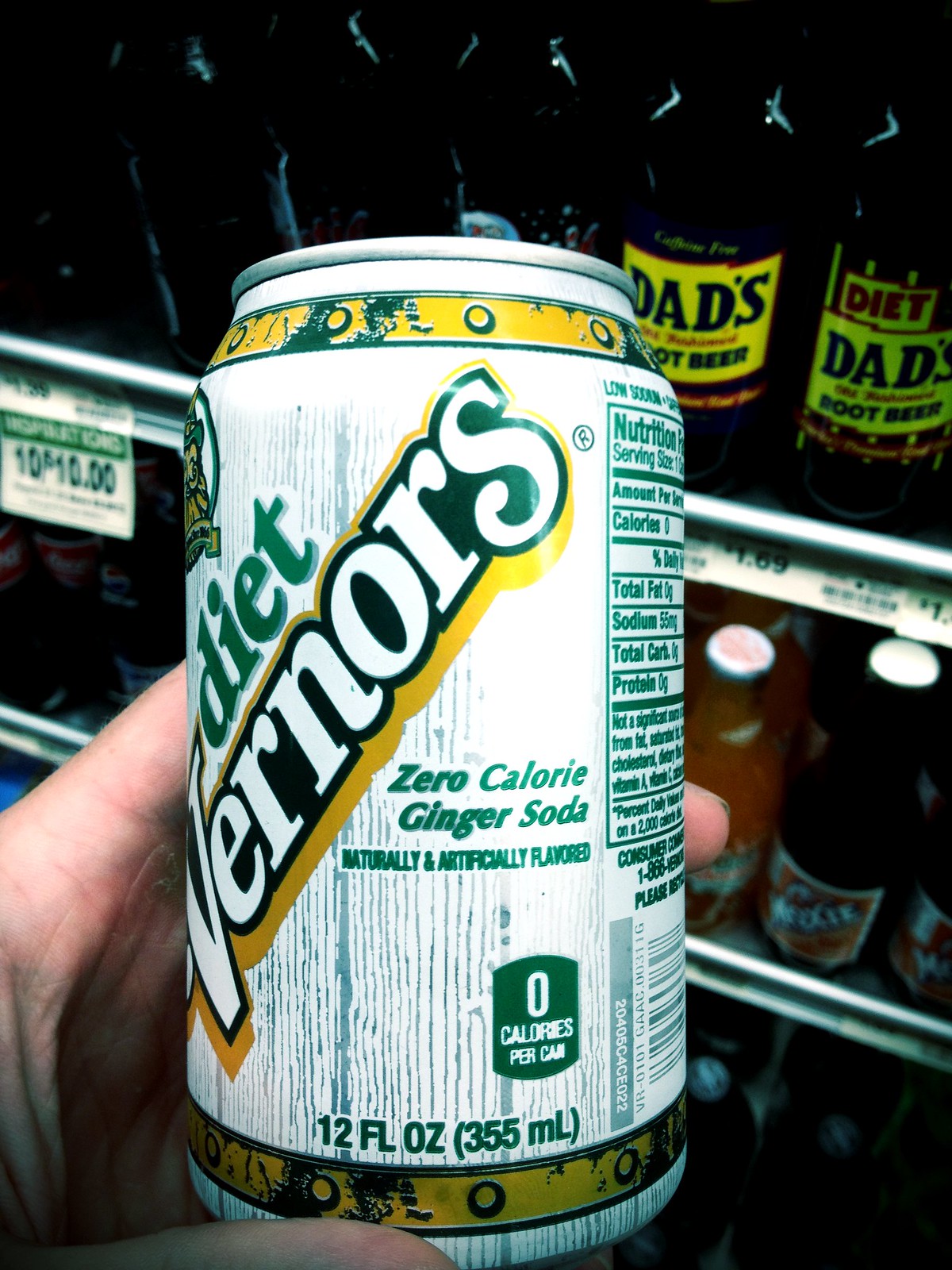A hand holds a can of Vernors Diet Ginger Soda against a white wooden background. The can, predominantly yellow at the top transitioning to green, features the text: "Diet Vernors Zero Calorie Ginger Soda, Naturally and Artificially Flavored." The bottom right displays "Zero Calories Per Can" in white text. Other beverages, including Dad's Root Beer with its orange and black label, are visible on a shelf in the background.